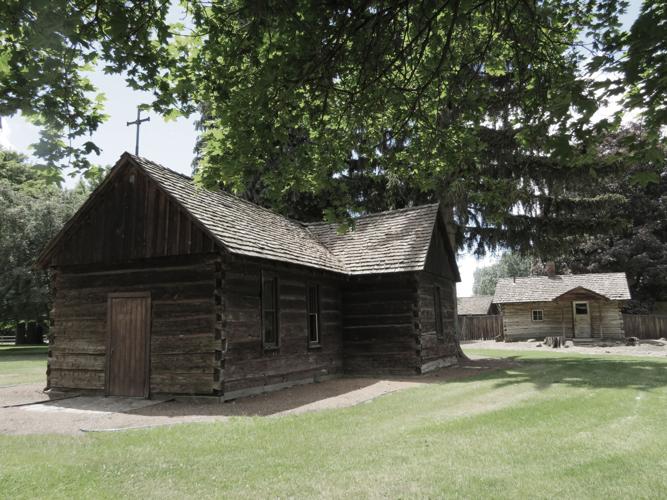This photograph captures a serene scene of an old, dark brown log cabin, potentially a former church, as indicated by the cross perched atop its pitched roof. The cabin, seemingly over a century old, stands as the focal point amidst a lush setting of green grass and towering trees that enclose it, complemented by pale blue sky peeping through the foliage. To the rear and right side of the image, there's a lighter-colored log cabin with a white door and a small covered porch. Both buildings give off a colonial-era vibe, indicating their age and historical significance. The tranquil environment, devoid of additional structures or traffic, evokes a sense of peaceful seclusion, suggesting a remote woodland locale. Additionally, a subtle detail of a power line can be seen in the background, hinting at the blend of old charm with traces of modernity.